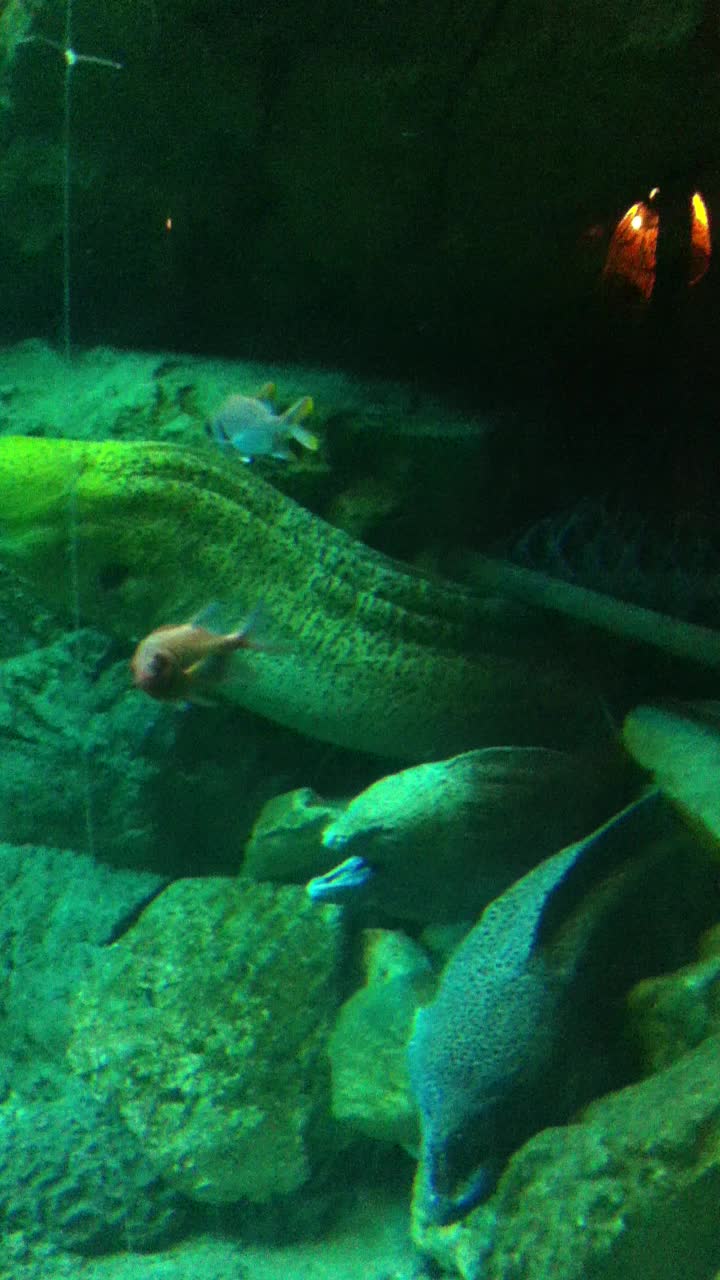The image depicts an underwater scene, likely from an aquarium, displaying a dark, moody atmosphere with a dark green hue dominating the upper part of the water. Dim light filters through the water on the upper right side, casting a subtle glow. A fishing line-like object extends down into the water. The seafloor is littered with large rocks covered in green algae and camouflaging an eel among them. Several fish populate the scene, including a bluish-colored fish, an orange or reddish fish, and multiple eels with varying colors, some with their mouths open and others closed. The eels have long, slender bodies, blending seamlessly with the rocks. One eel, in particular, is indistinguishable from the rock due to its camouflage. In addition to the eels, there are other fish present, one of which has prominent black eyes. The rocks and the entire scene exude a blend of green and dark green colors, contributing to the mysterious underwater ambiance.